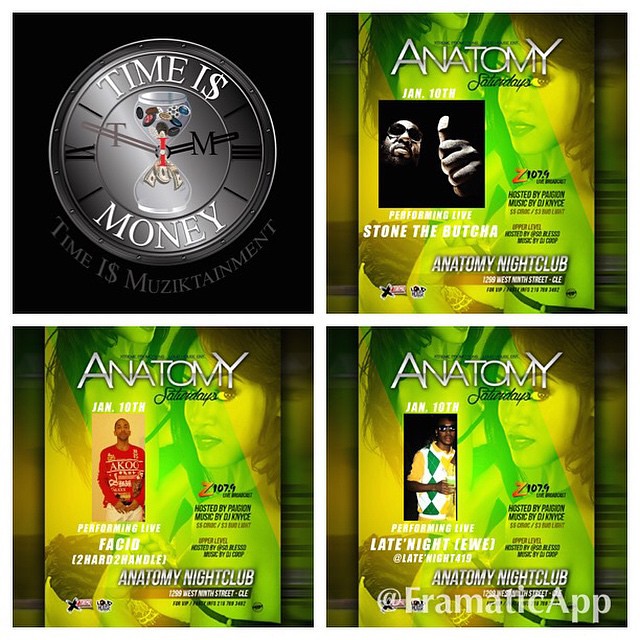The image consists of a four-image grid showcasing promotional materials and a thematic logo. The top left image features a black box containing a gray timepiece with the phrase "Time is Money," where the 'S' in 'Money' is replaced by a dollar sign. Inside this box, there's an hourglass filled with small clocks at the top, trickling down into dollar bills at the bottom, symbolizing the value of time. 

In contrast, the top right image is a vibrant club promotion flyer titled "Anatomy Saturdays," depicting a girl overlaid in green and a man with a black background, only his face is visible, peering out, identified as “Stone the Butcher,” set to perform live. Similar flyers appear in the bottom two images. The bottom left flyer features a man in a red sweater, labeled as "Facet Too Hard to Handle," while the bottom right shows a man in a green and yellow jersey, identified as “Late Night Uwu.” All the flyers share a consistent theme with the green and yellow color scheme, the date of January 10th, and venue information for the "Anatomy" nightclub at the bottom.